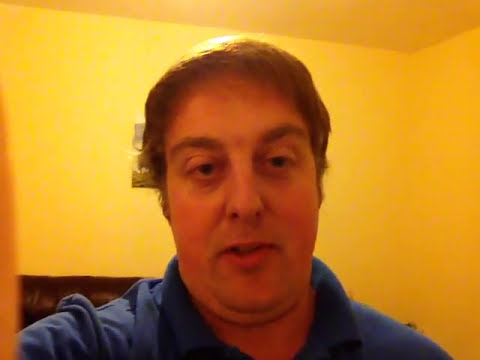The image captures a close-up view of a middle-aged white man, who appears to be taking a selfie. He has short to medium-length blonde hair and is wearing a blue collared shirt. His mouth is open slightly, and his eyes, though hard to discern due to the low lighting, are directed slightly below the camera lens. The room has an orange-yellow glow, with walls and ceiling painted in matching hues, and there’s a noticeable light source directly above him, casting a reflective glow on his hair. The background is largely obscured by his presence, but some details are visible: a partially visible picture frame or artwork peeks out just above his right shoulder, and a corner of an off-white drywall to the right. A brown leather sofa is also faintly visible behind him. The left side of the image is partially obscured, possibly by his thumb or another object, as he seems to be adjusting the camera.